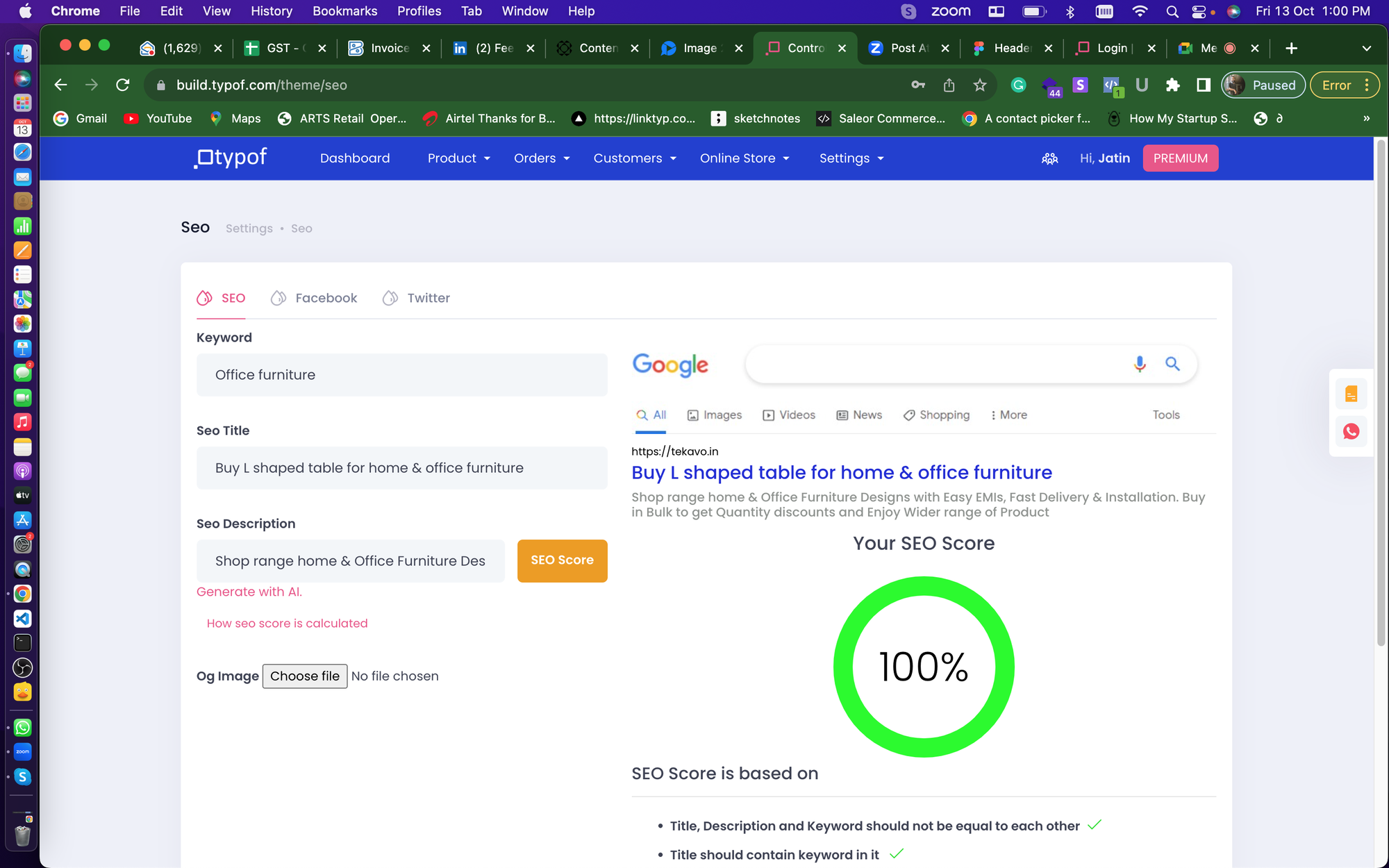This image captures a screenshot of a web browser, with the current tab displaying a page from the site "www.dypof.com/theme/SEO." In the top left corner of the window, the Apple logo is visible, indicating the use of a Mac. To the right of the Apple logo, the word "Chrome" is displayed, signifying the use of the Google Chrome browser. The browser's menu bar is fully visible, listing options for File, Edit, View, History, Bookmarks, Profiles, Tab, Window, and Help.

Below the menu bar, several open tabs are discernible, showing a busy browsing session. The primary content of the page centers around the website's dashboard interface. Various sections such as Dashboard, Products, Orders, Customers, Online Store, and Settings are accessible. A user is logged in and has navigated to an SEO analysis section of the site. The screen proudly shows an SEO score of 100%, indicating excellent search engine optimization for the site reviewed.